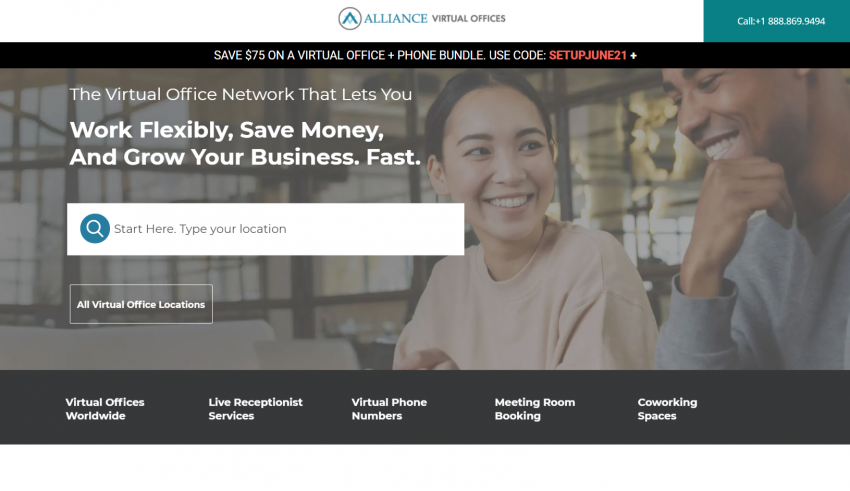The image appears to be a screenshot of a webpage that could be viewed on either a computer or a smartphone device, presented in a left-to-right horizontal layout. 

At the top left corner, there is a logo featuring a small circle in gray, with a teal 'A' icon inside. To the right of the logo, the brand name "Alliance" is written in teal, followed by "Virtual Offices" in black. 

On the upper right corner, there is a dark teal green rectangular box displaying a contact number in white text. Below this, a long black rectangular box contains the text "Save $75 on a virtual office phone bundle. Use code SETUPJUNE21," with the promotional code highlighted in red. A small white plus sign appears next to the text.

The background of the image displays a photo of a man and a woman engaged in conversation, both smiling. Superimposed on the background image is the text "The virtual office network that lets you," followed by "work flexibly, save money, and grow your business" in bold white text.

Beneath this, there is a white search box with a magnifying glass icon and the prompt "Start here, type your location." Next to it, there is another clickable box for browsing "All virtual office locations."

At the bottom of the image, a light black or dark gray bar lists services in white text: "Virtual offices worldwide," "Live receptionist services," "Virtual phone numbers," "Meeting room booking," and "Coworking spaces."